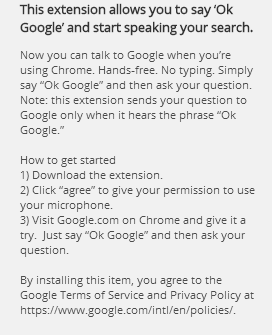The image depicts a pop-up information box on a website screen. The box is a vertical rectangle with a light gray background and dark-colored font. At the top of the box, a bolded sentence reads: "This extension allows you to say, 'Okay Google,' and start speaking your search." 

Beneath this header is a detailed description followed by a set of instructions for setting up voice activation for Google search. The initial blurb explains that users can talk to Google hands-free with Chrome by simply saying, "Okay Google," to initiate their query. It also notes that the extension sends your question to Google only when the phrase "Okay Google" is detected.

The setup instructions are as follows:
1. Download the extension.
2. Click 'Agree' and give permission to use your microphone.
3. Visit google.com on Chrome and give it a try. Simply say, "Okay Google," and ask your question.

At the bottom, there is a brief privacy statement indicating that by installing the extension, users agree to Google's privacy terms.